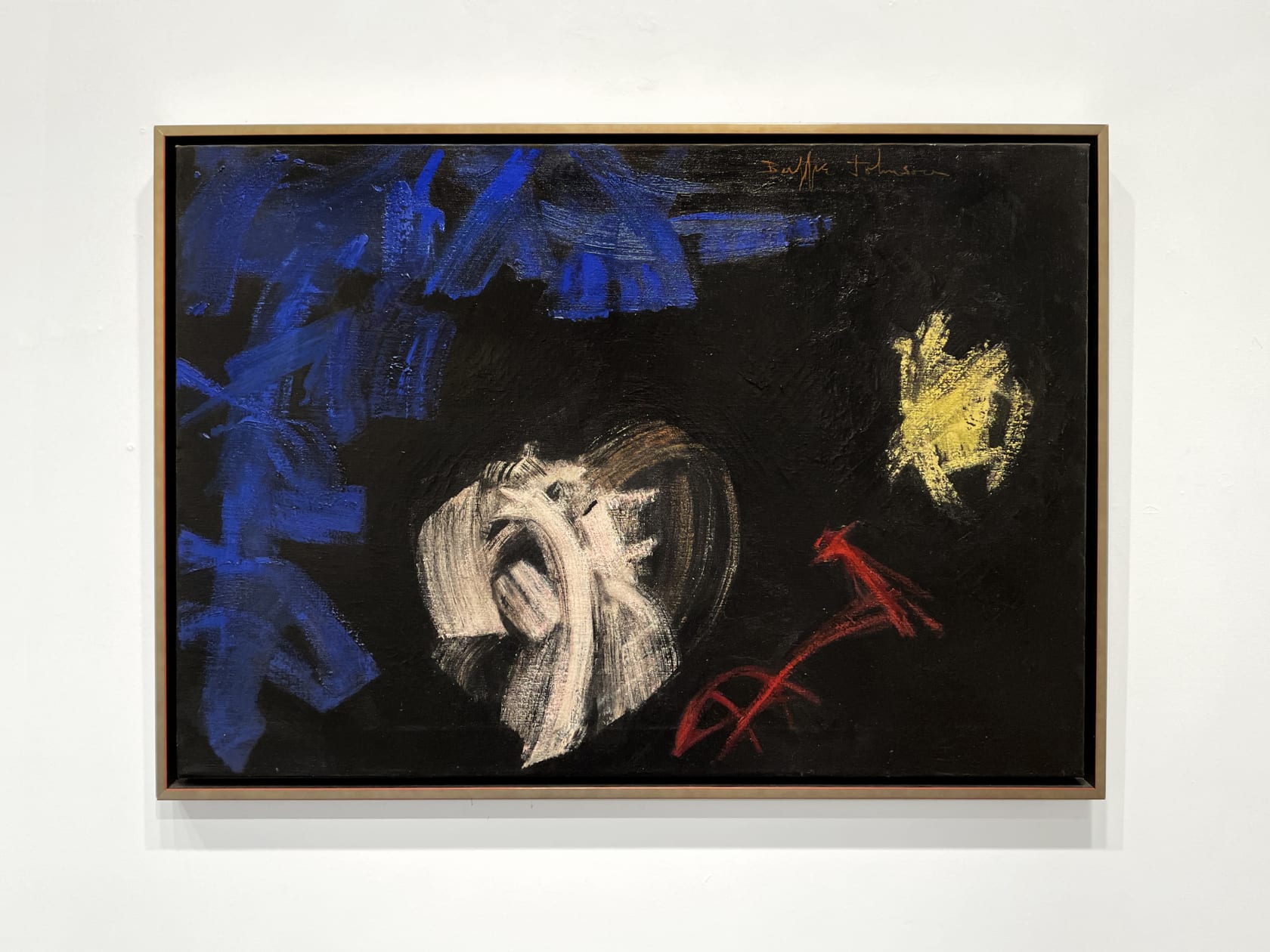The image is a full-color photograph of an artistic piece, square in shape, framed by a thick, faint blue border and an outer physical wood frame with a lighter brown hue casting a shadow below. The artwork itself is displayed on a black canvas or chalkboard. It features various colored chalk lines: large, sweeping blue marks positioned across the top left and extending downward; swirly white marks occupying the lower middle; thin red lines in the lower right; and splotchy yellow swirls near the middle right. The composition's design evokes a sense of abstract or possibly Asian influence. An artist's signature is visible in the upper right-hand corner, likely reading "something Johnson" or perhaps "Toberson," adding a personal touch to the creative display. The piece is hung against a soft white wall, accentuating its vibrant yet subtle details.